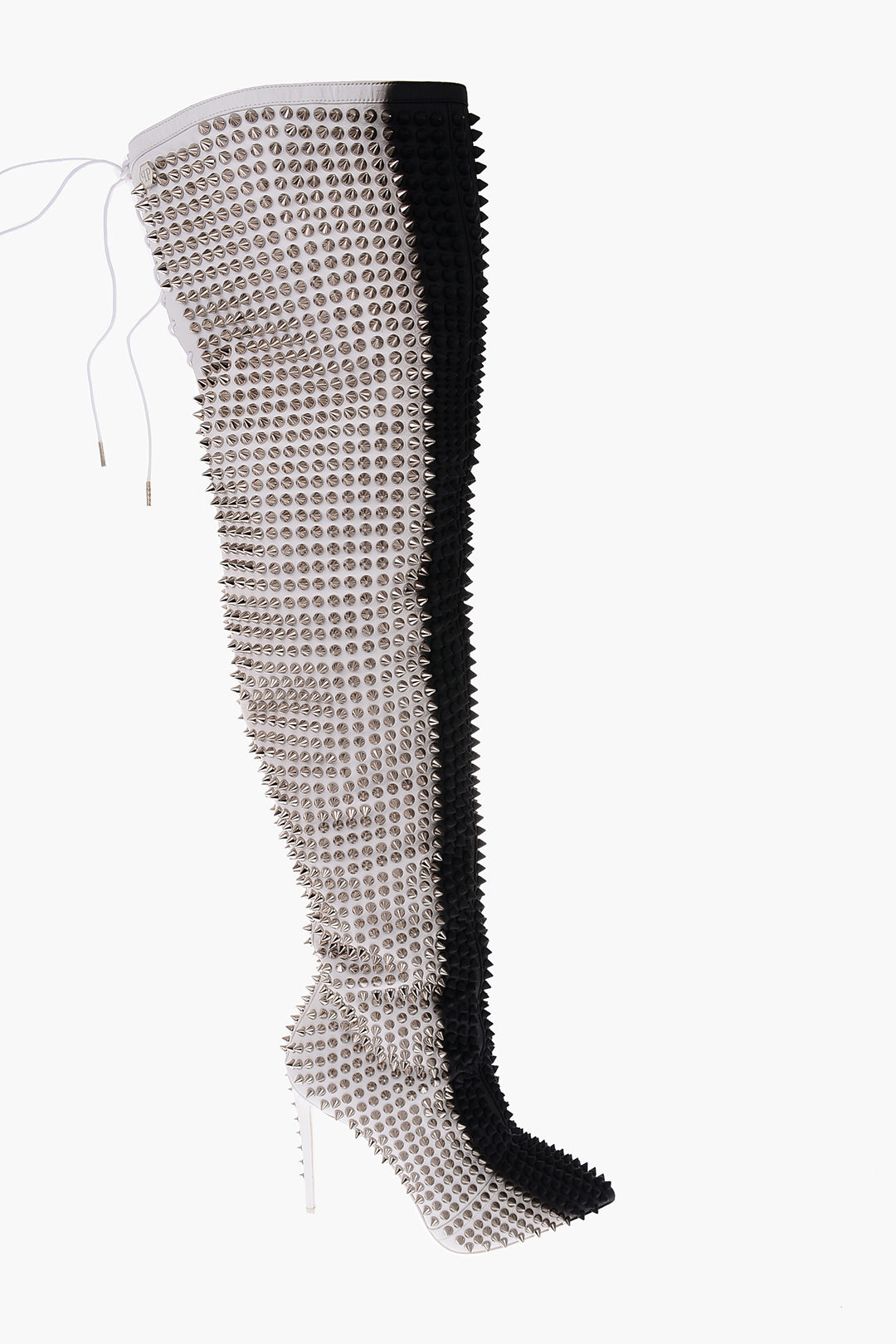The image showcases a digital photograph of a single high-heeled boot set against a stark white background. The boot, which appears to be about two feet tall, extends up to the thigh of the wearer and features a striking combination of black and white colors. The majority of the boot is covered in silver spiked studs, including a prominent four to five-inch stiletto heel also adorned with spikes. The boot has brown and white laces that dangle from its front, adding to its intricate design. Additionally, the photo features a noticeable black shadow cast behind the boot, highlighting its imposing presence.